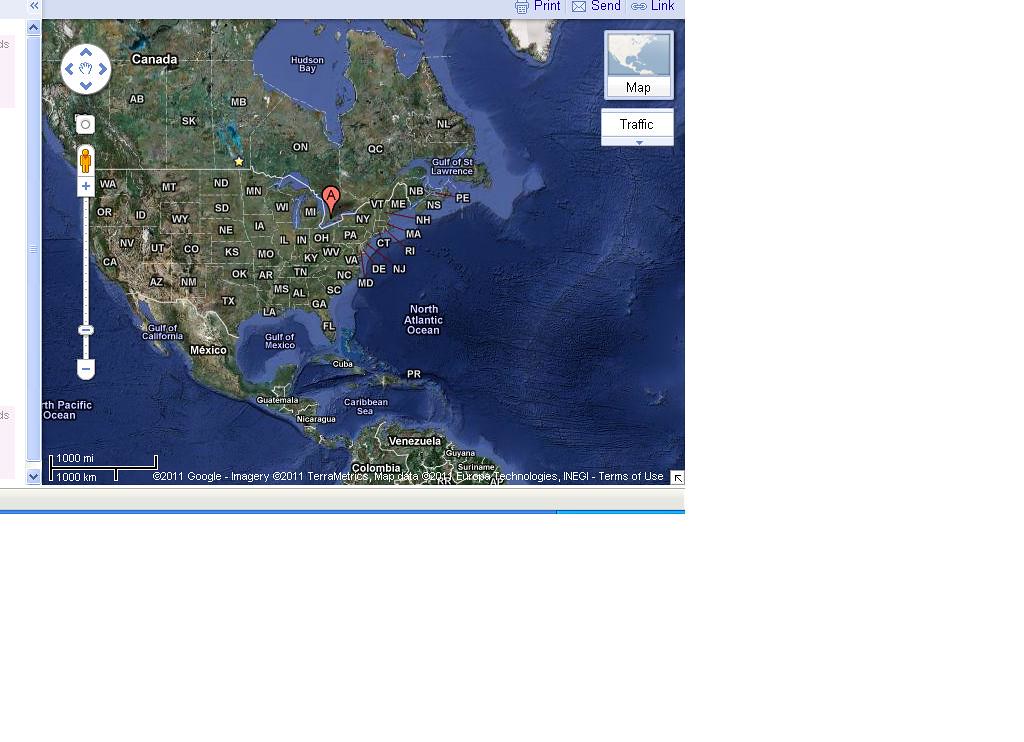A screenshotted image of a detailed map encompassing North America and portions of South America, prominently featuring the United States, Canada, Mexico, and the northern tip of South America, including countries like Venezuela, Colombia, Guyana, and Suriname. The map is highly zoomed out, showing a broad view with clear labels for geographical features such as the Caribbean Sea, Hudson Bay, Gulf of Mexico, and Gulf of California. Island details include Cuba and Puerto Rico. For Canada, all provinces are labeled, and there's a marked point labeled 'A' on the Canadian side near Ontario, suggesting a location like the Niagara Falls area. The map also displays a scale of 1000 miles and 1000 kilometers for distance measurement. The screen capture includes a blue-bordered interface with black text reading "Print", "Send", "Link" alongside their respective icons, alongside a white background with cropped window elements and a directional circle indicating north, south, east, and west. At the bottom, it is noted as "Copyright 2011 Google Imagery 2011 Terrametrics Map Data."